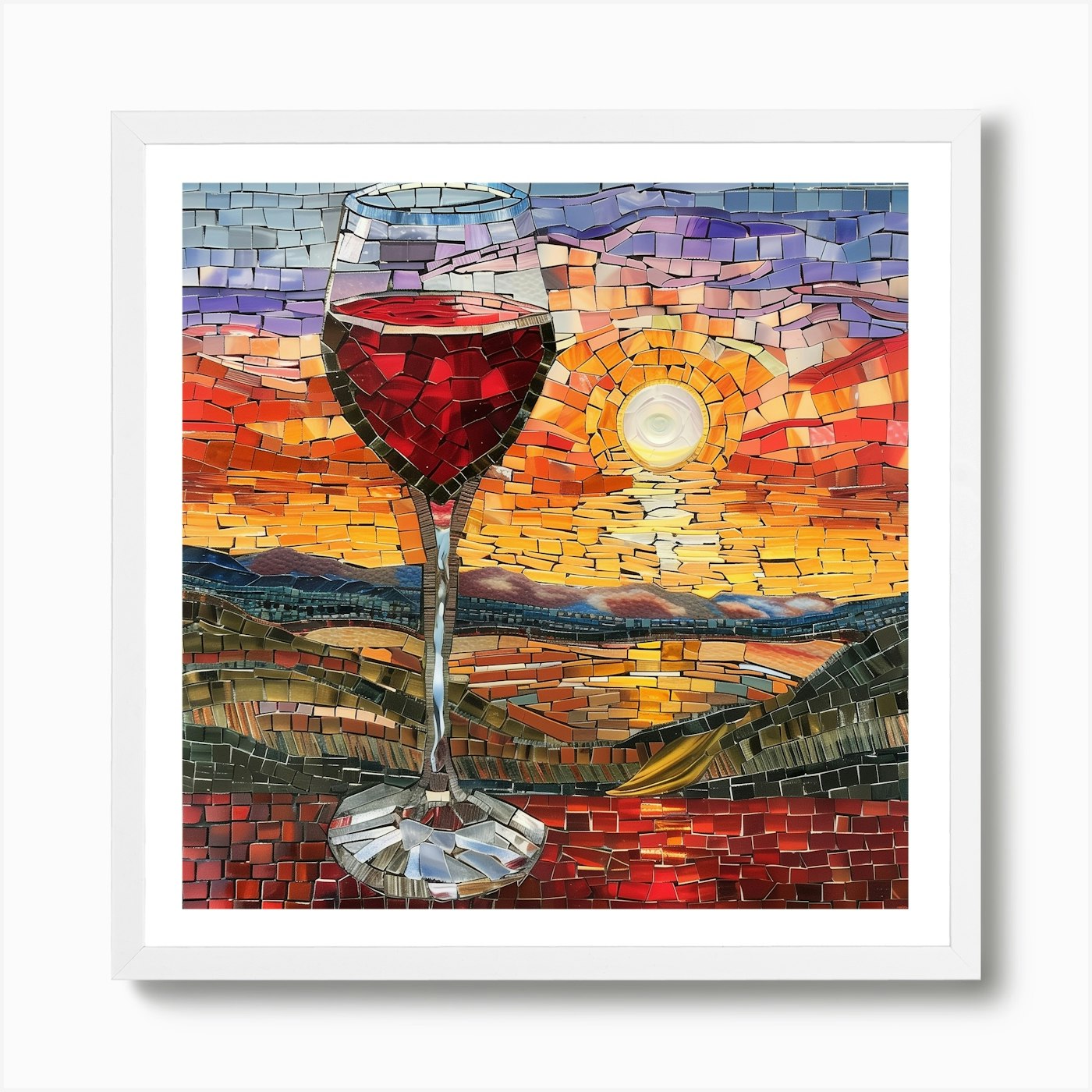This detailed mosaic artwork, framed in light gray with a white mat, hangs against an all-white wall, creating a stunning visual impact. The mosaic features a wine glass poised on a red mosaic shelf on the left side of the image. The glass, crafted from silver tiles, is filled halfway with a rich red liquid. The foreground of the image portrays green hills, implying a serene, hilly landscape, with what seems to be a body of water reflecting the descending sun. The scene is vivid, transitioning from light blue tiles at the top, morphing seamlessly into a purple and pink-hued sky. As it descends, the mosaic breathes life with reds, oranges, and yellows, highlighting a glowing white sun positioned to the right of the wine glass. The play of colors and intricate tile work captures the essence of a tranquil sunset, underscoring the wine glass as a focal point amidst this picturesque setting.